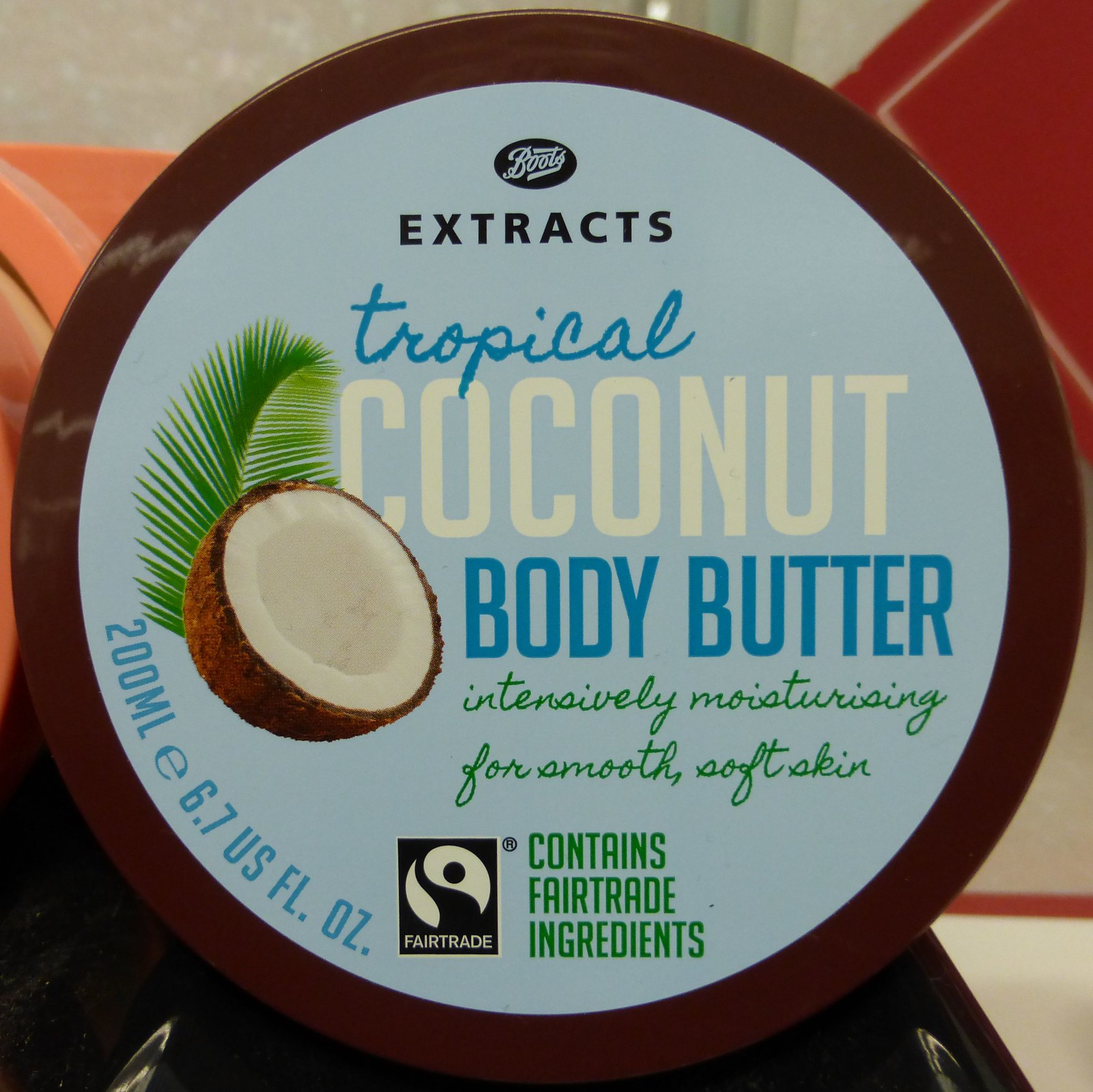This image captures the top view of a circular container of Boots Extracts Tropical Coconut Body Butter. The container edge is brown and its lid features a sky-blue background. Centralized at the top within a black oval logo is the text "Boots" in white, under which "Extracts" is printed in black capital letters. Below this, "Tropical" appears in medium blue cursive, followed by "Coconut" in white capital letters, and "Body Butter" in blue capital letters. The phrase "Intensely Moisturizing for Smooth Soft Skin" is inscribed in green cursive beneath. Towards the lower part of the lid, "Contains Fairtrade ingredients" is prominently stated in green capital letters accompanied by the Fairtrade logo, which is a black and white symbol of a person waving inside a circle with the word "Fairtrade" underneath. Next to the word "Coconut" lies an image of a palm leaf and a halved coconut. Near the 7-8 o'clock position on the lid, the measurement "200 milliliters e 6.7 US fluid ounces" is displayed, indicating the product’s volume. This richly detailed lid presentation emphasizes the fair trade certification and the product’s purpose to provide intense moisture for smooth, soft skin.